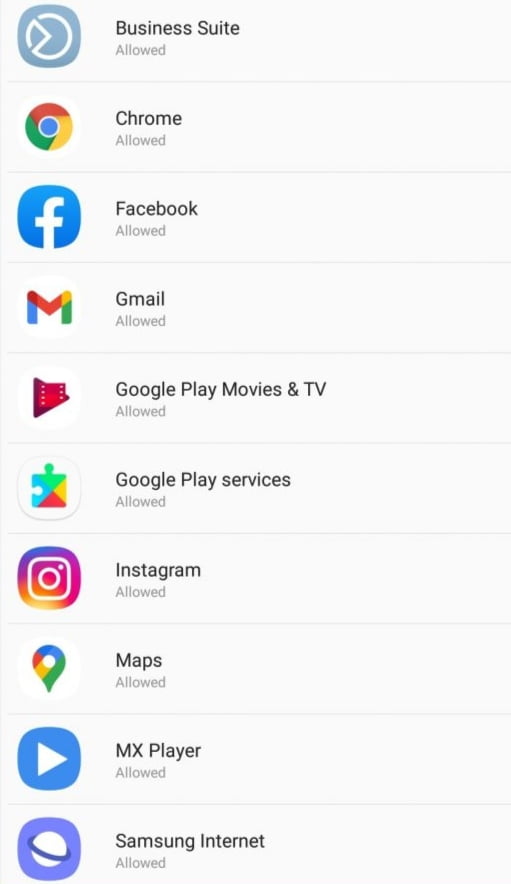The image features a gray background displaying a vertical list of different apps. Each app entry is separated by a slightly darker gray line, ensuring clear distinction between them. Positioned to the left of each app name is a corresponding icon. From top to bottom, the labeled apps and their respective status 'allowed' include:

1. **Business Suite** - with a gray symbol featuring a white circle intersected by a 90-degree angle on the left side.
2. **Chrome** - represented by its iconic red, yellow, green, and blue circular logo.
3. **Facebook** - denoted by its recognizable blue square with a white 'F' in the center.
4. **Gmail** - symbolized by a vibrant, multicolored 'M'.
5. **Google Play Movies and TV** - presumed to have its standard icon, although the description does not specify.
6. **Google Play Services** - presumed to have its default icon, though specifics are not detailed.
7. **Instagram** - identified by the purple gradient camera logo.
8. **Maps** - inferred to have its typical location pin icon, though not specified.
9. **MX Player** - likely shown with its standard blue triangle logo, not specifically described.
10. **Samsung Internet** - presumably depicted with its usual purple globe icon, not explicitly outlined in the description.

Overall, the captions provided are highly descriptive, detailing both visual elements and the organizational structure of the app list.